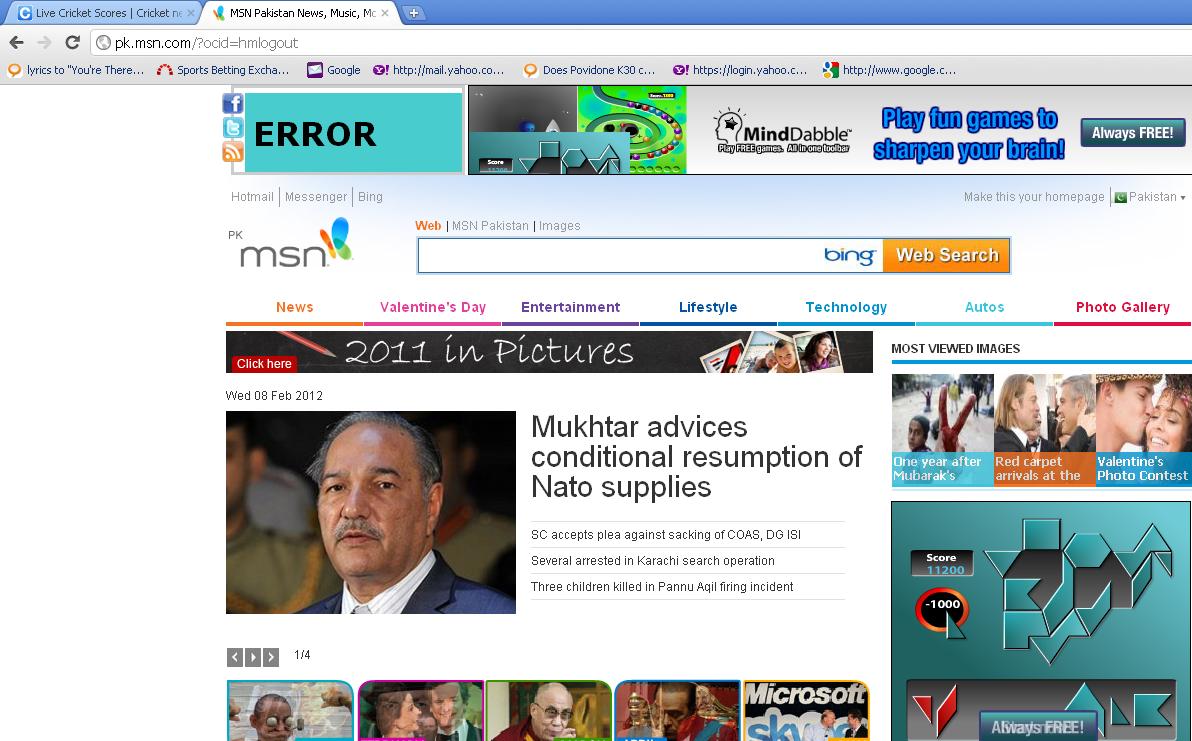A screenshot of a desktop web browser displaying two open tabs on the left side of the screen. The first tab is labeled "Live Cricket Scores," while the second tab, which is currently active, is partially visible and reads "MSN Pakistan News Music." The browser shows a search bar just below the tab row, followed by a horizontal grey bar filled with bookmarks. 

The body of the active website features a predominantly white background. At the top, there is a large advertisement with a blue square on the left that says "Error" and three vertically aligned social media icons (Facebook, Tumblr, and RSS) next to it. Adjacent to this ad is another advertisement with the text "Play Fun Games to Sharpen Your Brain Always Free Mind Dabble," accompanied by a small game thumbnail.

Below these ads, the MSN logo is positioned in the top left corner, and to its right, there is a search bar with the word "Bing" on the far right and an orange "Web Search" button. A row of categories follows, including "News," "Valentine's Day," "Entertainment," "Lifestyle," "Technology," "Autos," and "Photo Gallery." Beneath this row, a banner reads "2011 in Pictures," and further down, articles are listed. The first article features a large thumbnail image of a man on the left, with the story's caption displayed to the right.